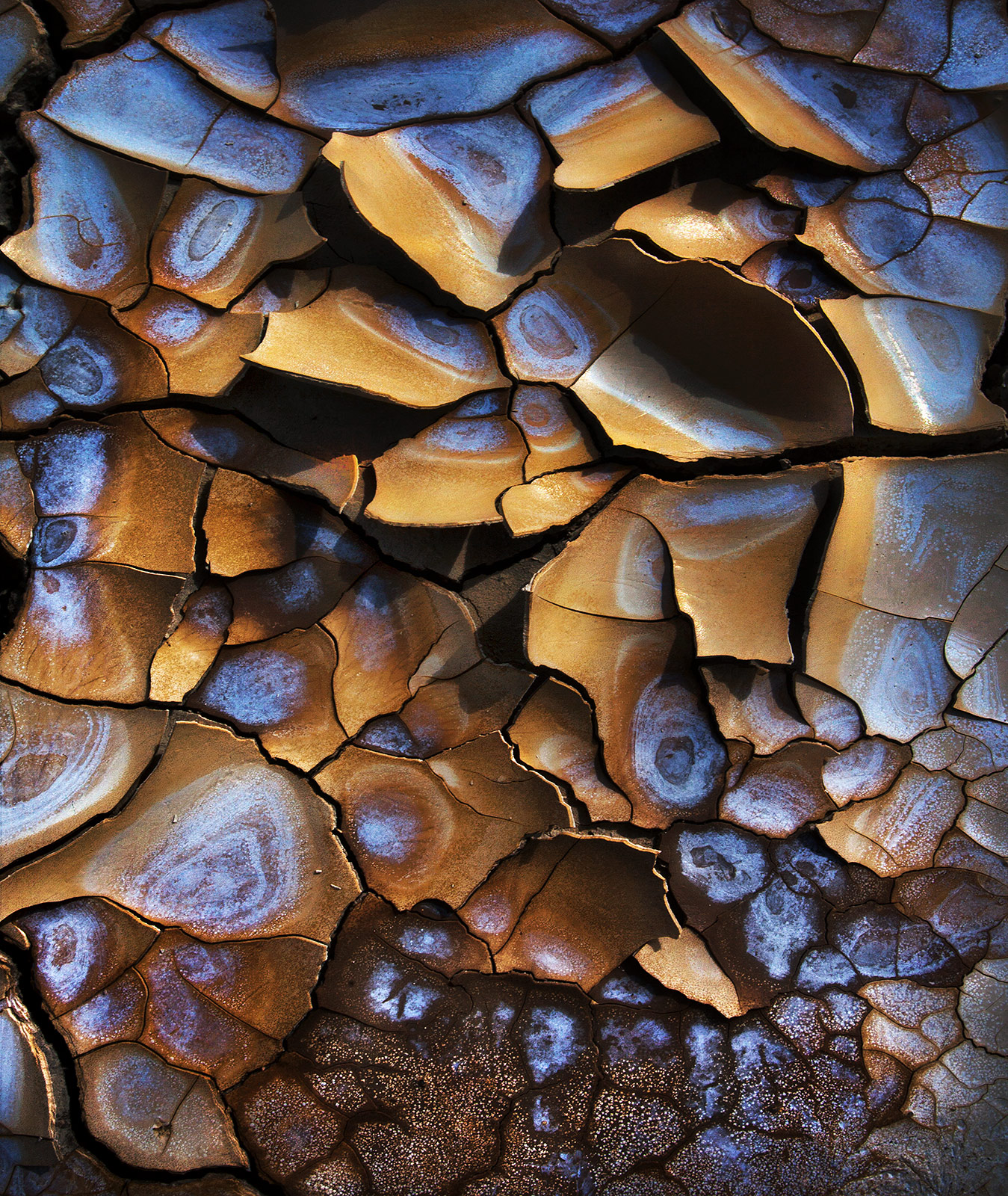In this color image, we see a highly detailed, segmented, craggy surface resembling a dried creek bed or the intricate texture of wood grain. The background is predominantly brown, interspersed with distinct white concentric circles or chalky rings that give it an almost fogged or mildewed appearance. The segments appear broken and fragmented, fitting together like random puzzle pieces. Notably, the bottom right section of the image is darker and speckled with tiny white dots, indicating a varied texture. The photo lacks a sense of scale, making it ambiguous whether we are observing a macro shot of a natural object, possibly wood or rocks, or a bird's eye view of a landscape. This surface might be reminiscent of weathered rocks on a beach, marked by water and sand.